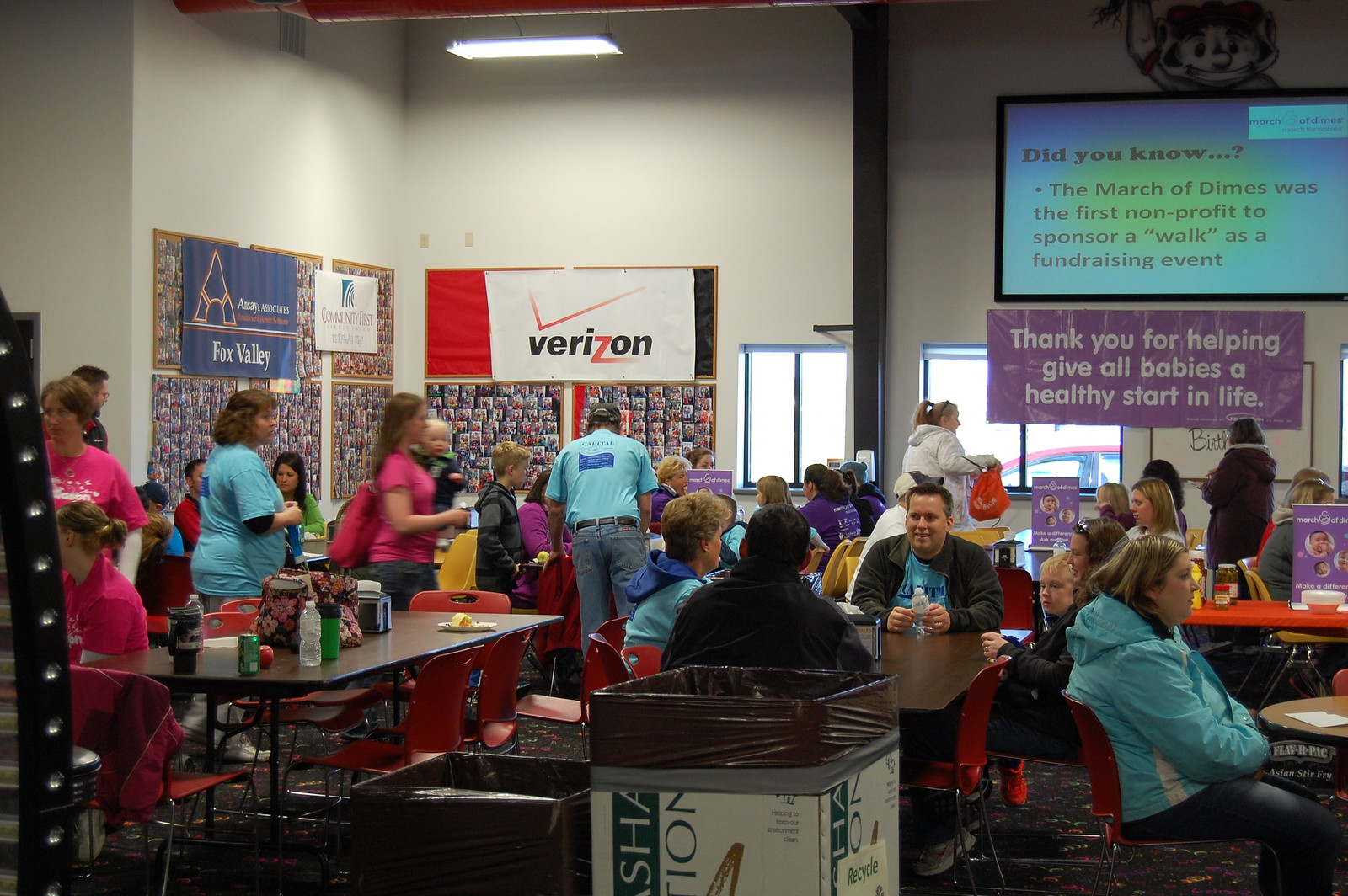The image depicts a bustling restaurant setting with several wooden tables, each surrounded by people engaged in conversation. The tables and chairs are centrally positioned, and a few individuals are seen moving around the space. The floor features a patterned carpet, adding to the cozy ambiance. Prominently displayed on the walls are various advertisements and posters, mostly dedicated to the March of Dimes charity. Notable among these is a sign stating, "Did you know the March of Dimes was the first non-profit to sponsor a walk as a fundraiser event?" Additionally, there's a message thanking patrons for "helping give all babies a healthy start in life." Other visible ads include a Verizon advertisement. The predominant colors in the image include shades of white, red, blue, pink, brown, orange, black, and gray. A centrally placed trash can can also be seen. The indoor scene, likely captured during the day, seems to be set at a charity event, as evidenced by the themed decorations and signage.